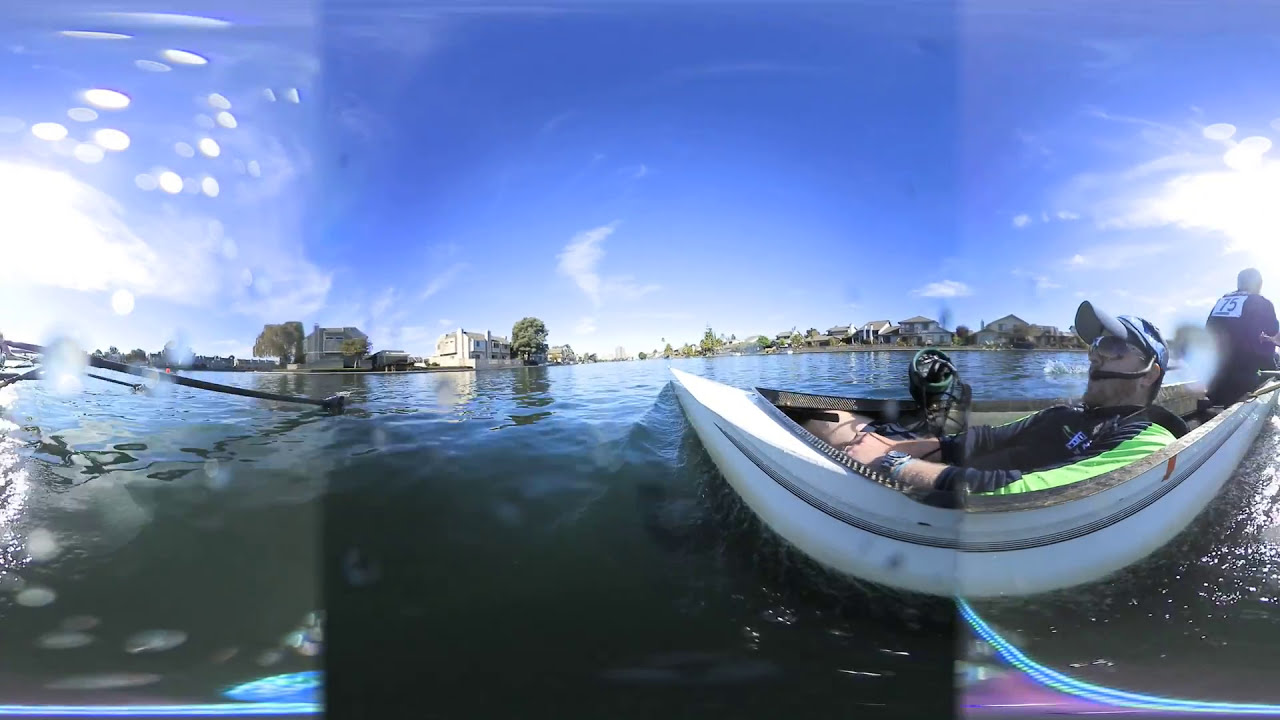This slightly distorted outdoor photo, likely taken with an unconventional lens, captures a unique scene on the water. The main focus is a white boat, which appears arch-shaped due to the distortion. Centrally placed, a man is lying back in the front of the boat, wearing a black sweatshirt with neon green stripes, a headset, sunglasses, and a black and blue baseball cap. This gentleman seems to be the captain or pacing the team on a racing canoe styled after those used by Harvard or Yale. Another man is visible in the background, sporting a shirt with the number 15 and complementing the figurehead of the boat. The waters reflect the clear blue sky with very few clouds, and the scene is framed by distant buildings against the horizon. On the far side, oars from a competing boat can be seen, adding context to the race. The image is divided into different blocks of clarity, with the left and right edges blurred, emphasizing the central figures amid the river's reflective surface.